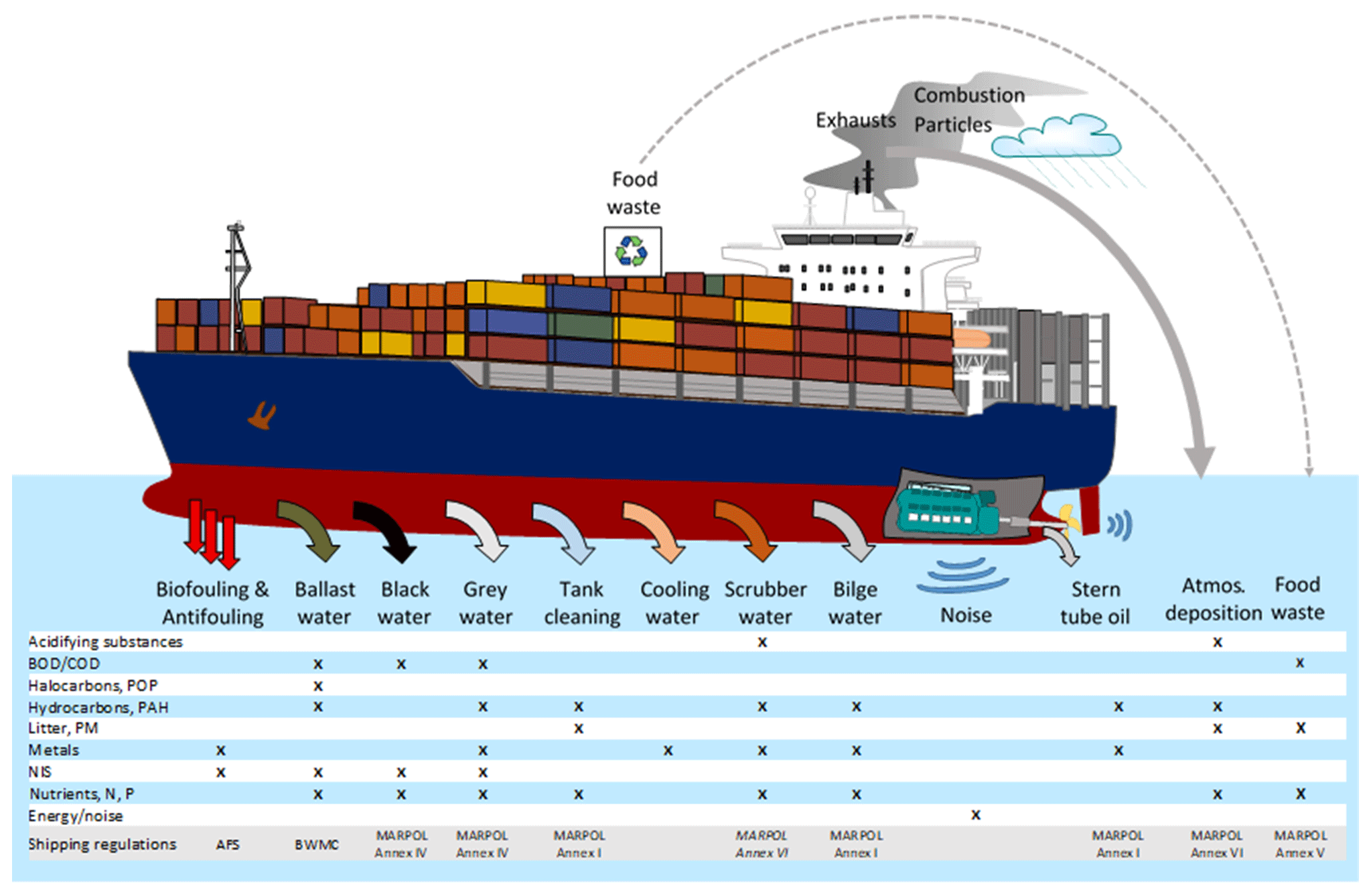This is a digitally created illustration featuring a cargo ship in vivid detail, primarily showcasing the various types of pollution and waste it produces. The ship, with blue sides and a red bottom beneath the waterline, carries rectangular 3D containers. Above the ship, clouds and labels like food waste, exhaust, and combustion particles indicate airborne emissions. Surrounding the ship, arrows highlight various pollutants such as biofouling, antifouling, ballast water, black water, gray water, tank cleaning water, cooling water, scrubbing water, bilge water, noise, and stern tube oil. Below, there is a detailed chart listing these pollutants alongside the consequences of their release—such as metals from gray water and acidifying substances from scrubbing water. Additionally, the chart includes headings like cooling water, tank cleaning, noise, and atmospheric deposition, arranged in columns, with corresponding effects like BOD/COD, litter, and PM in rows. Shipping regulations, mentioned at the bottom, include names like Marpol Annex VI, indicating what they regulate. The illustration uses a palette of colors including dark blue, red, pink, light blue, beige, gray, light gray, dark green, yellow, orange, and black, with the ship positioned above the water and the chart below, providing a comprehensive overview of maritime pollution and its regulatory context.